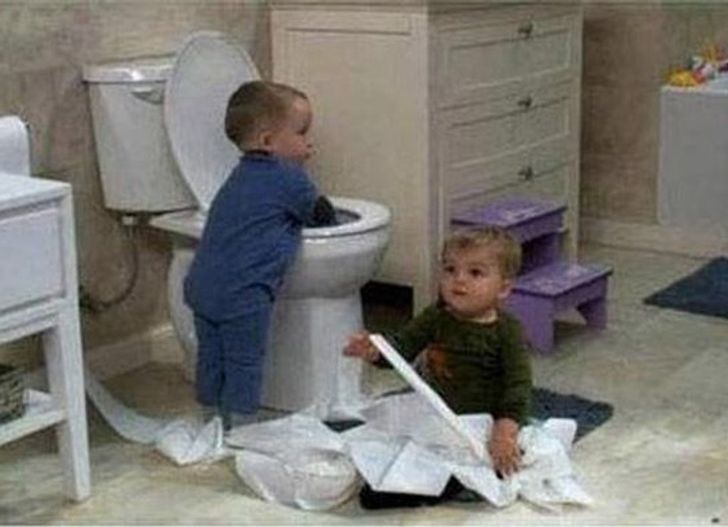In this slightly fuzzy photograph, two toddlers, seemingly under a year old, are creating chaotic yet adorable mischief in a bathroom. One toddler, dressed in a green shirt, has unraveled the toilet tissue, which now covers his lap and is strewn all across the floor. He is sitting on one of the two blue rugs, playing with the tissue while looking upward. The floor beneath is a whitish hue. Beside him stands a cream-colored chest of drawers with a purple step stool in front. The second toddler, dressed in a blue outfit consisting of a top and matching pants, is standing near an open white toilet with his hands submersed in the water, though his gaze is focused off to the side. Behind him, a white table can be faintly discerned through the blur. The background features something indistinct and white on the back wall, adding to the domestic ambiance of the scene.